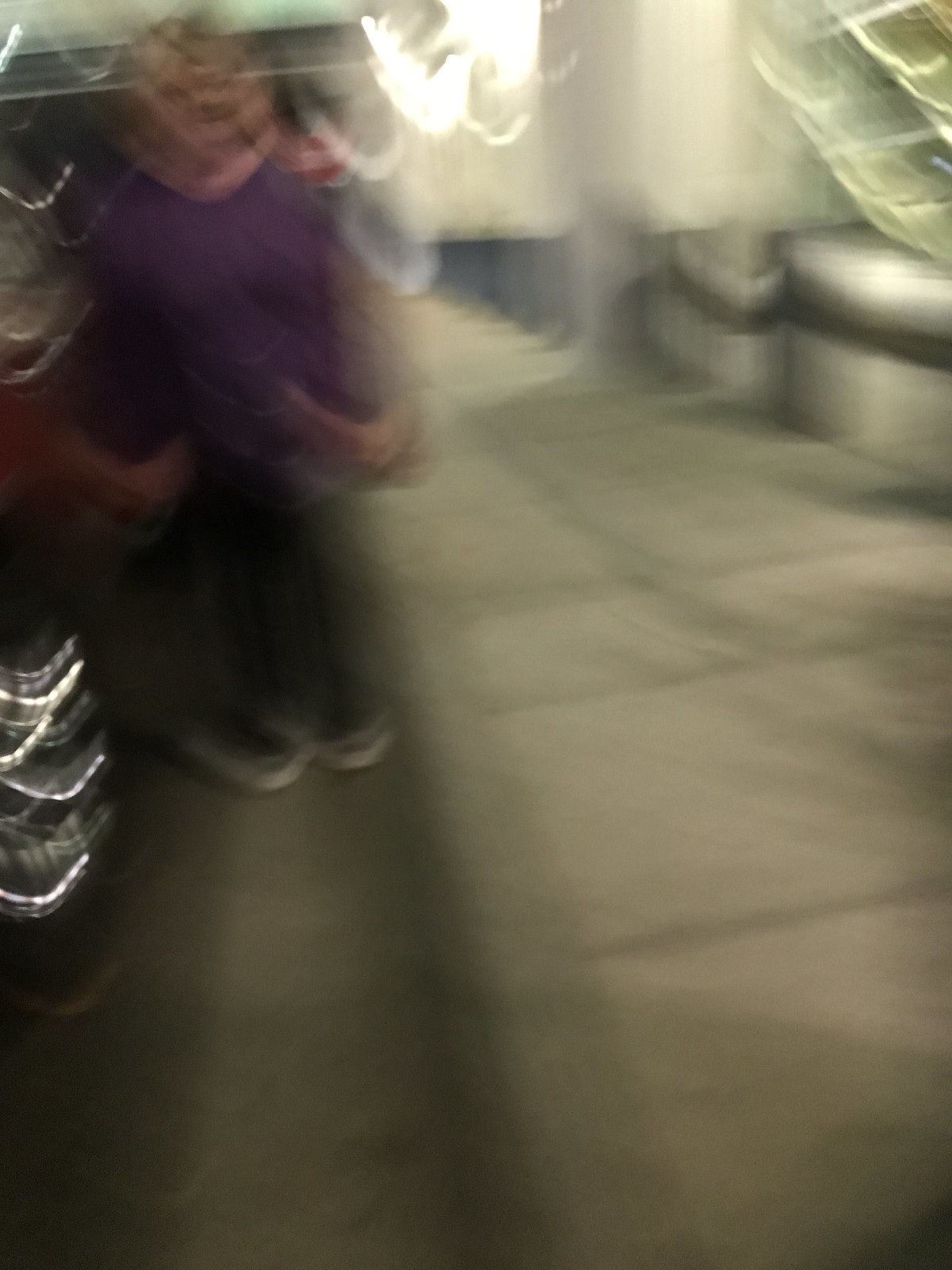This color photograph, taken in portrait orientation, is significantly blurred, making it challenging to discern precise details. The foreground features a hard-surfaced, gray floor. Further along this floor stands an individual wearing white shoes paired with dark pants and a long-sleeved purple shirt. The person's blonde hair is visible, though their face is distorted by the blur. To the left, a portion of another person's arm is visible. The room is brightly lit, with some objects on the floor adorned with string lights. Daylight filters in from ahead, illuminating walls and other indistinct structures within the room.